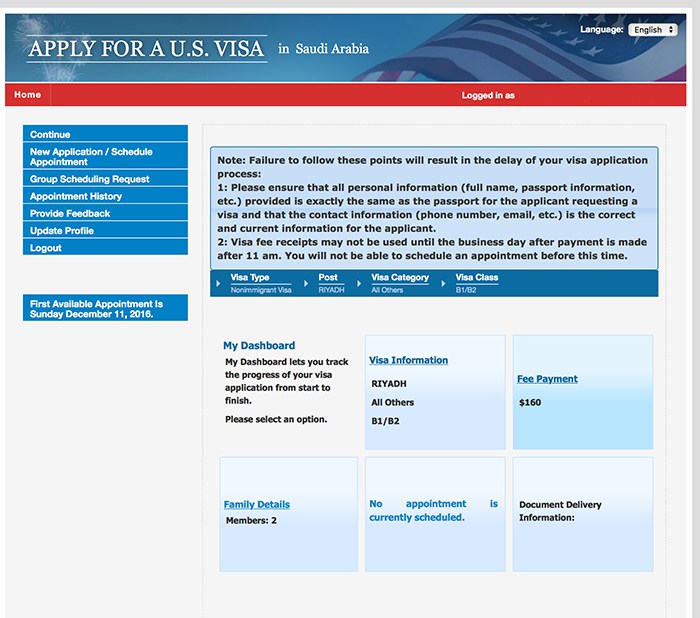**Detailed Caption:**

This is a detailed screenshot of a U.S. government website dedicated to visa applications specifically for Saudi Arabia. The header features a vivid U.S. flag and celebratory fireworks, creating a visually engaging entry point. Located in the upper right-hand corner, the language option is set to English by default. Just below this area, a prominent red navigation bar hosts several links such as "Home" and a placeholder for the user’s login status, which is currently not visible.

The left side of the page contains a vertical menu with a series of blue rectangular buttons stacked vertically, offering options like “Continue,” “New Application,” “Schedule Appointment,” “Group Scheduling Request,” “Appointment History,” “Provide Feedback,” “Update Profile,” and “Logout.” After navigating through a substantial amount of white space, the website informs the user that the first available appointment is on Sunday, December 11, 2016, highlighted against a blue background but not fashioned as a clickable button.

On the right side, a section begins with a header titled "Note," which warns that failing to comply with listed instructions will delay the visa application process. These instructions emphasize verifying all personal information and details regarding fees, visa types, categories, and classes. This is followed by an overview under "My Dashboard," which provides essential details such as "Visa Info," "Fee Payment ($160)," "Family Details (2 members)," and a notice stating that no appointments are currently scheduled. Information on document delivery is also displayed, underscoring that while no actions have been initiated yet, this is the centralized place for managing the entire visa application process.